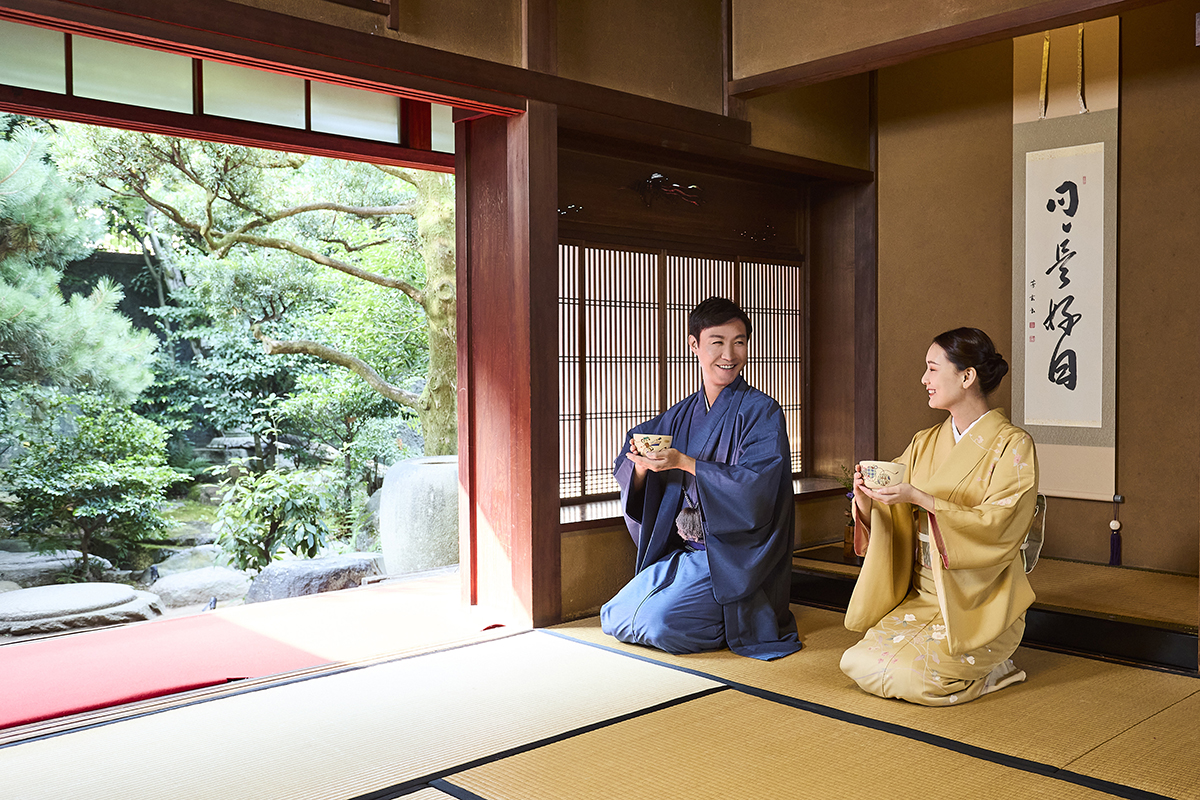In this captivating image, we see a serene moment shared between a man and a woman kneeling inside a traditional dojo, adorned in beautiful kimonos. Both individuals are positioned on the right side of the image, with the man on the left wearing a flowing blue kimono and the woman on his right adorned in a gold one, her dark hair elegantly styled in a bun. Each of them holds a small bowl in their hands, exchanging warm smiles that suggest a deep connection.

The dojo itself exudes a rich cultural ambiance, with beige mats trimmed in dark brown placed across the floor, and a large entryway on the left side of the image that opens up to reveal lush green trees outside. A vivid red rug lies at the top of the steps leading out to the greenery, adding a touch of color to the tranquil setting. In the background behind the couple, a vertical picture with Oriental characters adds to the authentic atmosphere, reminiscent of the peaceful settings often depicted in classic films like "Karate Kid" and conjures a sense of calm and tradition.